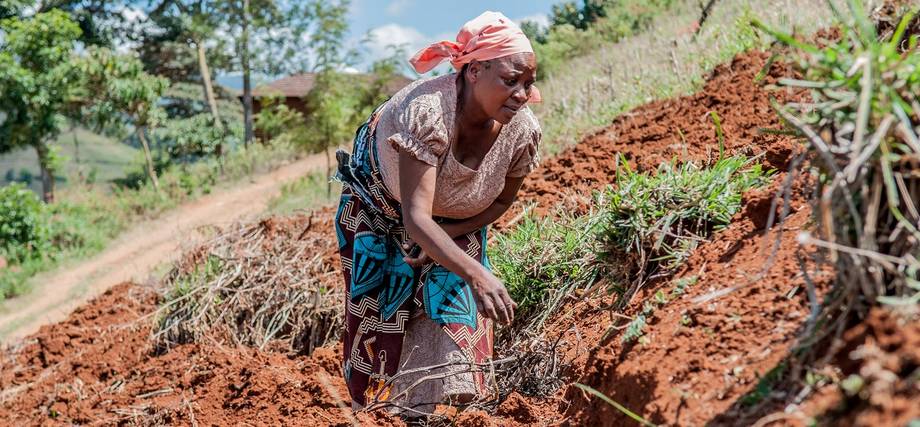The image depicts an older African-American woman working diligently in a sunny outdoor setting. She is bent over at the waist and appears to be either planting or weeding among freshly churned, rich brown dirt. She has brown skin and is adorned in traditional African attire, including a brown dress and a pink headscarf tied around her head. Additionally, a blue, brown, and white patterned cloth, possibly a quilt, is wrapped around her waist. The scene is set on a sloping hill featuring patches of lush green grass and various plants, including some that might be weeds. In the background, there is a line of diverse trees and green bushes, a dirt road leading up to a brown house, and a clear blue sky with some clouds, indicating a bright, sunny day.